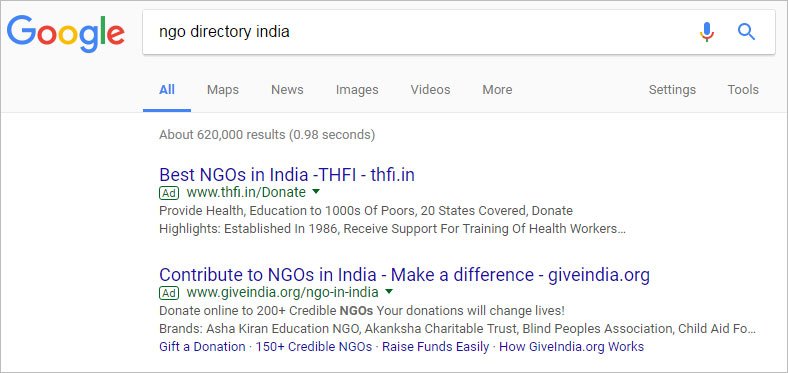**Detailed Screenshot Description:**

This image is a screenshot from Google search results. 

On the left-hand side of the search bar, the Google logo is prominently displayed. It consists of a dark blue "G," followed by a red "o," a yellow "o," a blue "g," a green "l," and a red "e." The logo stands out against a gray background.

In the URL bar, black text reads "NGO directory India."

Next to the URL bar, on the right, there are two icons. The first is a blue microphone with red sound waves emanating from it, and beneath it, a single green line. The second icon is a dark blue magnifying glass.

Above the search results are several tabs. The selected tab, labeled "All," is highlighted in blue with a blue line underneath it. The other tabs are "Maps," "News," "Images," "Videos," and "More," all in gray text. On the far right-hand side, there are options labeled "Settings" and "Tools."

Under this navigation bar, a white area contains search results. At the top, in dark gray text, it states there are approximately 620,000 results found in 0.98 seconds.

The first search result is a hyperlink with blue text: "Best NGOs in India - thfi - thfi.in." Below this, in green text, "Ad" is written, followed by a URL: "www.thfi.in/donate" along with a green rightward arrow. 

Accompanying this link, black text provides a brief description: "Provide health education to thousands in 20 states covered. Donate. Highlights: Established in 1986, receive support for training of health workers."

The final visible result also features blue hyperlinked text: "Contribute to NGOs in India - Make a Difference - giveindia.org." Next to it, in green text within a rectangle, is the word "Ad." The associated URL is "www.giveindia.org/NGO-in-India."

Below this URL, black text reads: "Donate online to 200+ credible NGOs." The term "NGOs" is bolded. The text continues: "Your donations will change lives!" 

Further details include: "Brands: ASHA, ASHA Kiran Education NGO, Akansha Charitable, Trust Blind People's Association, Child Aid for…", but the rest of the text is cut off.

This comprehensive description captures the visual elements and textual content found in the screenshot.